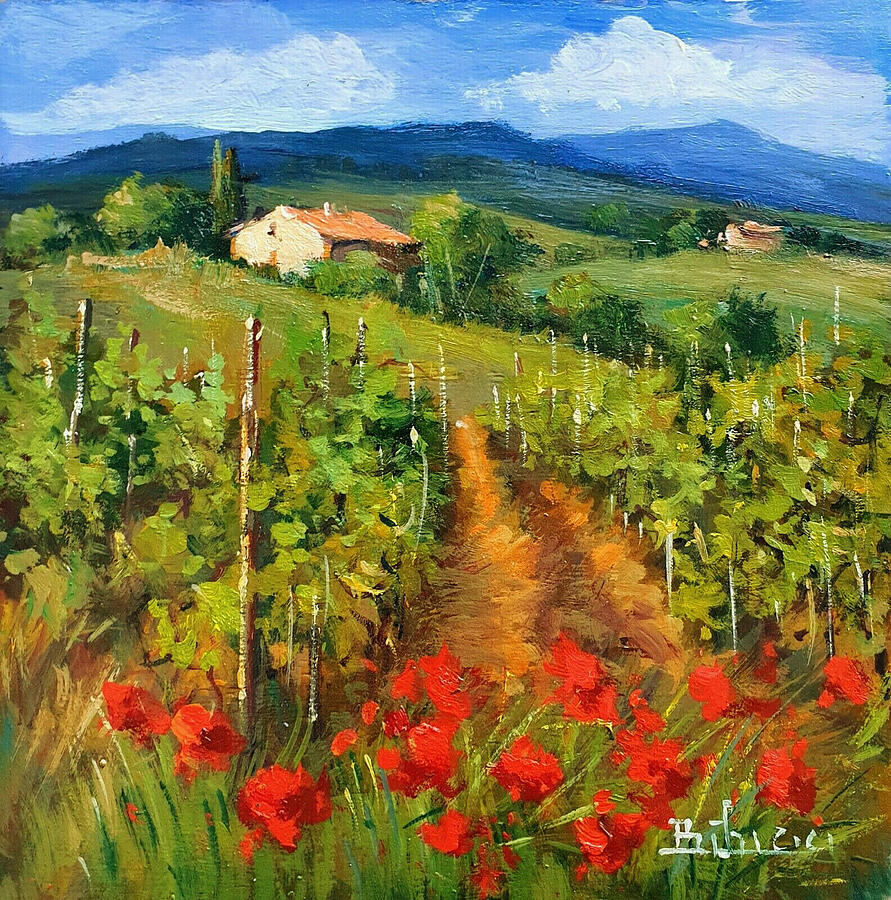This enchanting square artwork captures a serene landscape beneath a tranquil blue and white sky, featuring a mountain range painted in muted blues and grays with soft, delicate strokes. The scene unfolds from the bottom up, starting with a vibrant bed of red roses and high grass, transitioning seamlessly into rows of plants that appear to be cultivating vegetables or fruit. Nestled in the idyllic setting is a beige-colored, single-story home with a brown roof, adding a touch of warmth. In the distance, to the upper or lower right, another light beige structure, possibly a barn or another dwelling, can be glimpsed, its shape indistinct. The absence of livestock or human figures emphasizes the serene isolation of the scene. The artist, Babichi, has signed their name in white paint in the lower right corner, completing this picturesque composition.